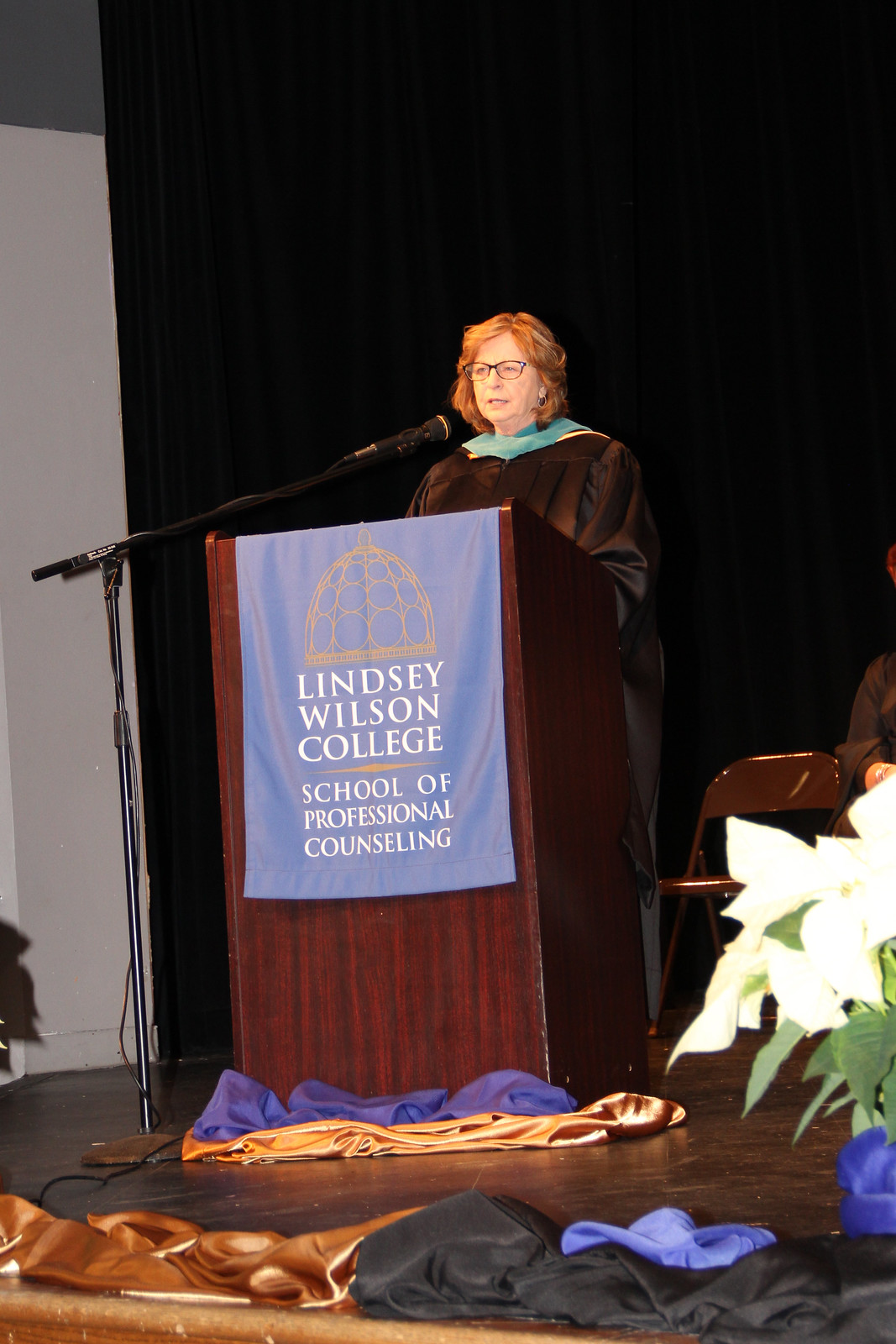The image captures a graduation ceremony at Lindsay Wilson College, specifically for the School of Professional Counseling. At the center, a distinguished older woman with dark glasses and striking red hair stands behind a dark wood podium. She is speaking into a well-positioned microphone at mouth level. She wears a traditional black graduation gown. The podium features a blue banner with a stylized cupola and the text "Lindsay Wilson College School of Professional Counseling." In front of the podium, a floral arrangement with white flowers and green foliage can be seen, along with draped fabrics in shades of gold, black, purple, blue, and bronze scattered on the brown wooden stage. The background is a simple black backdrop, partially revealing gray walls and metal chairs positioned for the event.